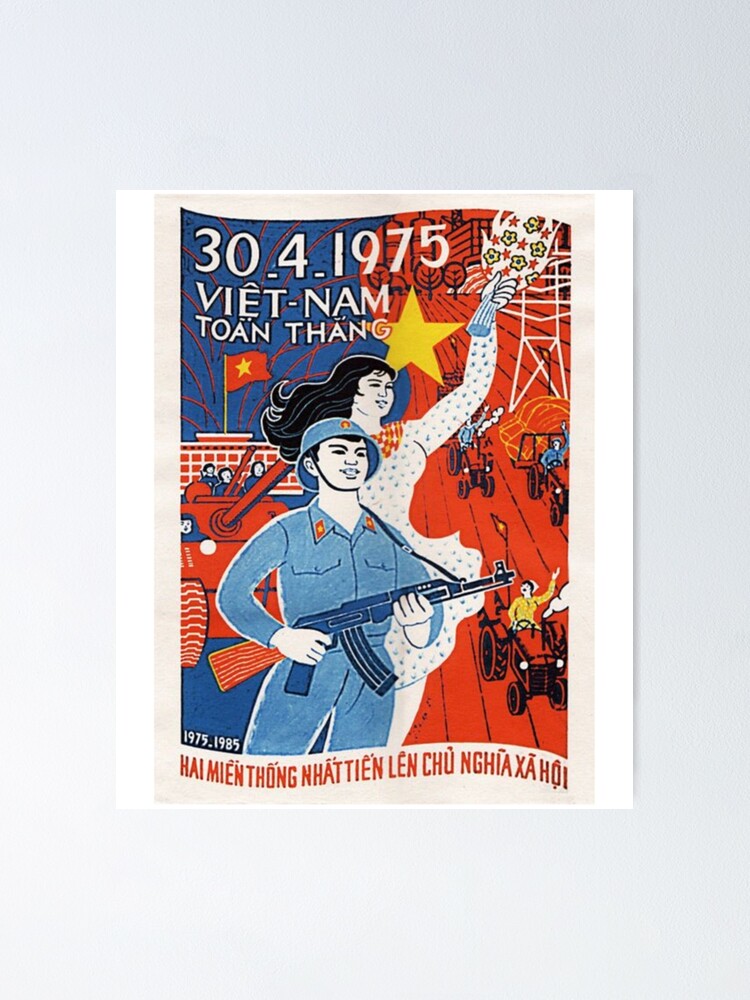This image captures a detailed close-up of a commemorative stamp, dated 30-4-1975, Vietnam. The central figure is a Chinese soldier dressed in cyan-blue attire, including a helmet and white gloves, holding a blue AK with an orange-brown stock, and looking to the right. Behind him stands a woman in a white dress adorned with blue polka dots, holding a blue-striped vase with yellow flowers and a white background featuring red stars. She wears a red and white striped bow tie. In the background to the left, a red tank occupied by individuals in dark blue is visible, along with a Vietnamese flag above a white building. To the right, people are driving a series of red, cyan-blue, dark blue, and yellow tractors, with white smoke billowing from the exhaust of the nearest one. The upper right corner features a white radio tower. The text at the bottom is in Vietnamese, mentioning the years 1975-1985, against a red background where the tractors are positioned. The stamp is placed on a beige piece of paper.